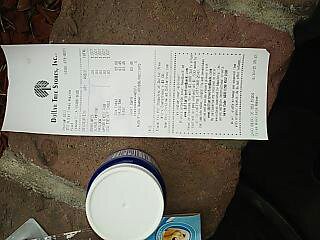This photograph captures a slightly blurry Dollar Tree store receipt positioned on a red brick surface. The receipt, though illegible except for the recognizable "Dollar Tree" logo, is filled with numerous lines of black text on a white, rectangular piece of paper. Adjacent to the receipt, there is a cylindrical plastic container with a white lid and a blue body. Additionally, some unclear plastic items are visible at the bottom of the image. Underneath the container, a blue piece of what appears to be part of a cardboard box or bag peeks out. The contrasting colors and the placement on the brick background create an interesting and layered visual composition.